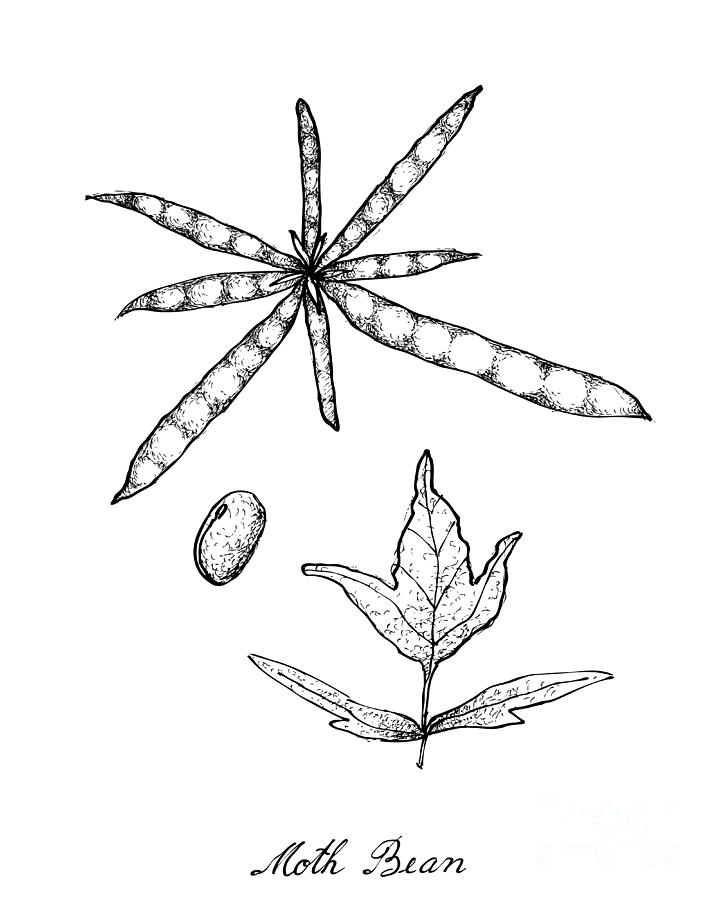This detailed black and white illustration, executed with pen and ink, portrays various parts of the moth bean plant arranged vertically. At the top, the drawing highlights a starfish-like structure, featuring eight extended pods radiating from a central point, each pod containing what resemble green peas or beans. Below this, the middle section showcases an oval-shaped bean or pod. At the bottom of the image, the detailed depiction shows a stalk with three leaves, the central leaf being the largest and most prominent, with three distinct points, while the two smaller, longitudinally shaped leaves each have two points. The entire drawing is meticulously shaded and labeled "Moth Bean" in elegant script at the bottom center, drawing attention to the different stages and parts of the plant.